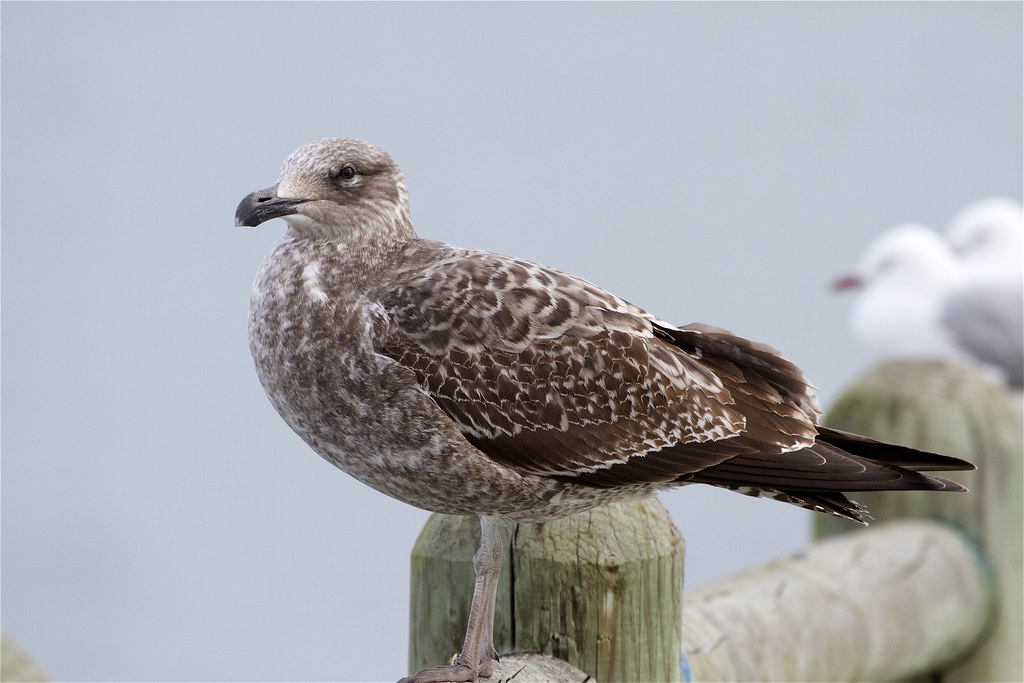In this outdoor daytime photo, a lone pigeon with light marble-brown feathers and darker brown wings is perched on a wooden fence. The pigeon faces to the left, its ashen beak pointing slightly forward, and has a frosted appearance on its light brown face. The background is a hazy blue, suggesting a foggy environment. To the right in the blurred background, two seagulls with white puffy feathers and gray wings can be seen, likely on the same wooden fence. This serene scene hints at a possibly coastal setting.